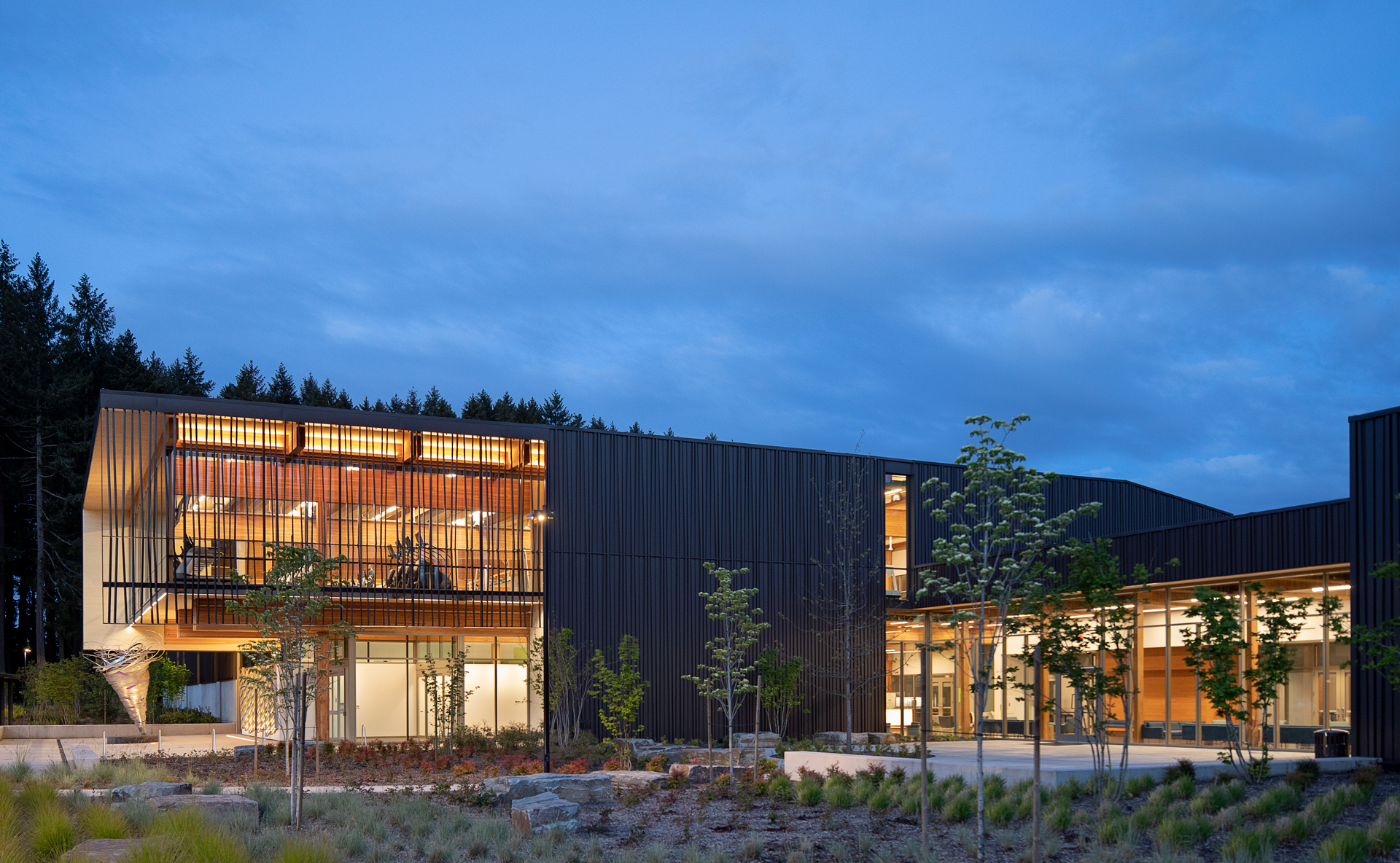In this outdoor early evening photograph, the scene is illuminated by both natural and artificial light, casting a soft, dusky glow. The sky, featuring some clouds, takes up most of the top portion of the square image, painting the setting with shades of light and dark blue indicating twilight. A row of pine trees lines the left side of the scene, adding a touch of natural greenery.

Dominating the image are two modern buildings, possibly part of a school campus, composed of large floor-to-ceiling windows that reveal glimpses of the illuminated interiors. The building on the left is a rectangular, two-story structure with dark sheet metal siding, extending from the center of the photo to the left. The right side of the image showcases the entrance of the second building, which appears to be connected to the first, extending from the mid-center to the right. 

Between these structures, the landscaping includes patches of light-colored dirt interspersed with young trees supported by stakes, small tufts of grass, and bushes, while the foreground features rocky dirt. The color palette of the photograph includes various shades of blue, green, brown, black, and off-white, creating a harmonious blend of natural and architectural elements.